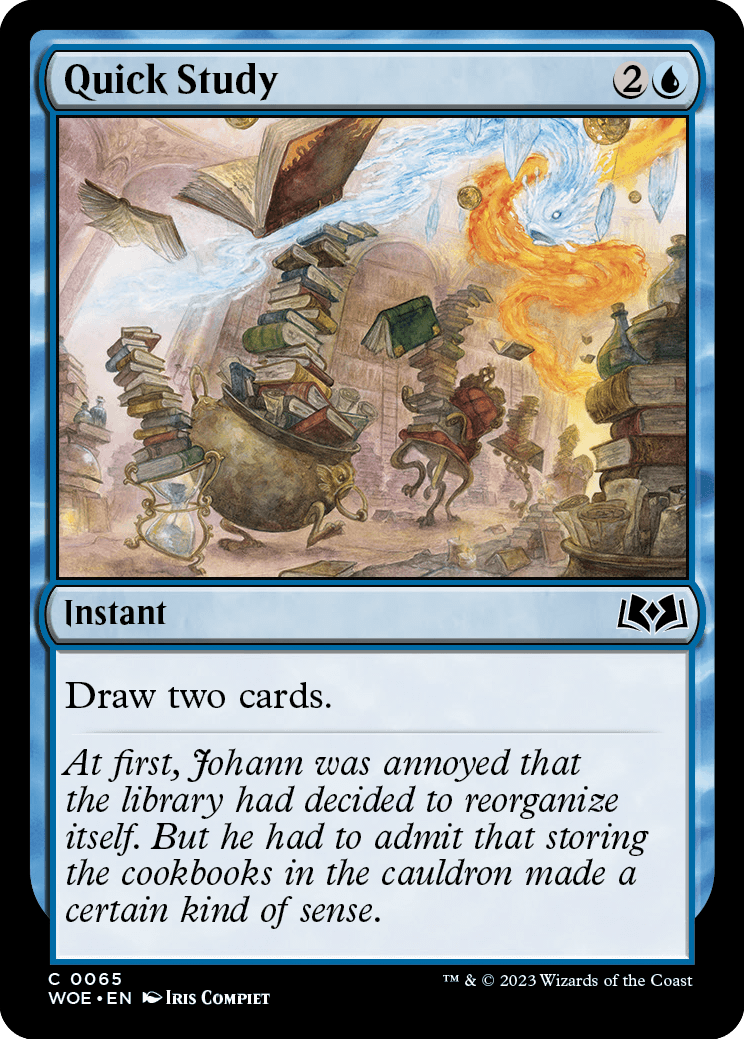An image of a Magic: The Gathering card titled "Quick Study" is featured. The card is bordered in blue, with a watery texture that adds a mystical ambiance. The central illustration is a chaotic yet captivating scene where books appear to defy gravity, flying and falling from the sky. Some books are balanced precariously on an hourglass, while a cauldron brims with a stack of volumes. Additionally, books are teetering atop a walking chair, contributing to the whimsical disorder. Positioned below the image, the card's type is denoted as "Instant," accompanied by an icon of a book on the right. The card's effect is succinctly described with the text, "Draw two cards." A flavor text beneath reads: "At first, Johan was annoyed that the library had decided to reorganize itself. But he had to admit that storing the cookbooks in the cauldron made a certain kind of sense."